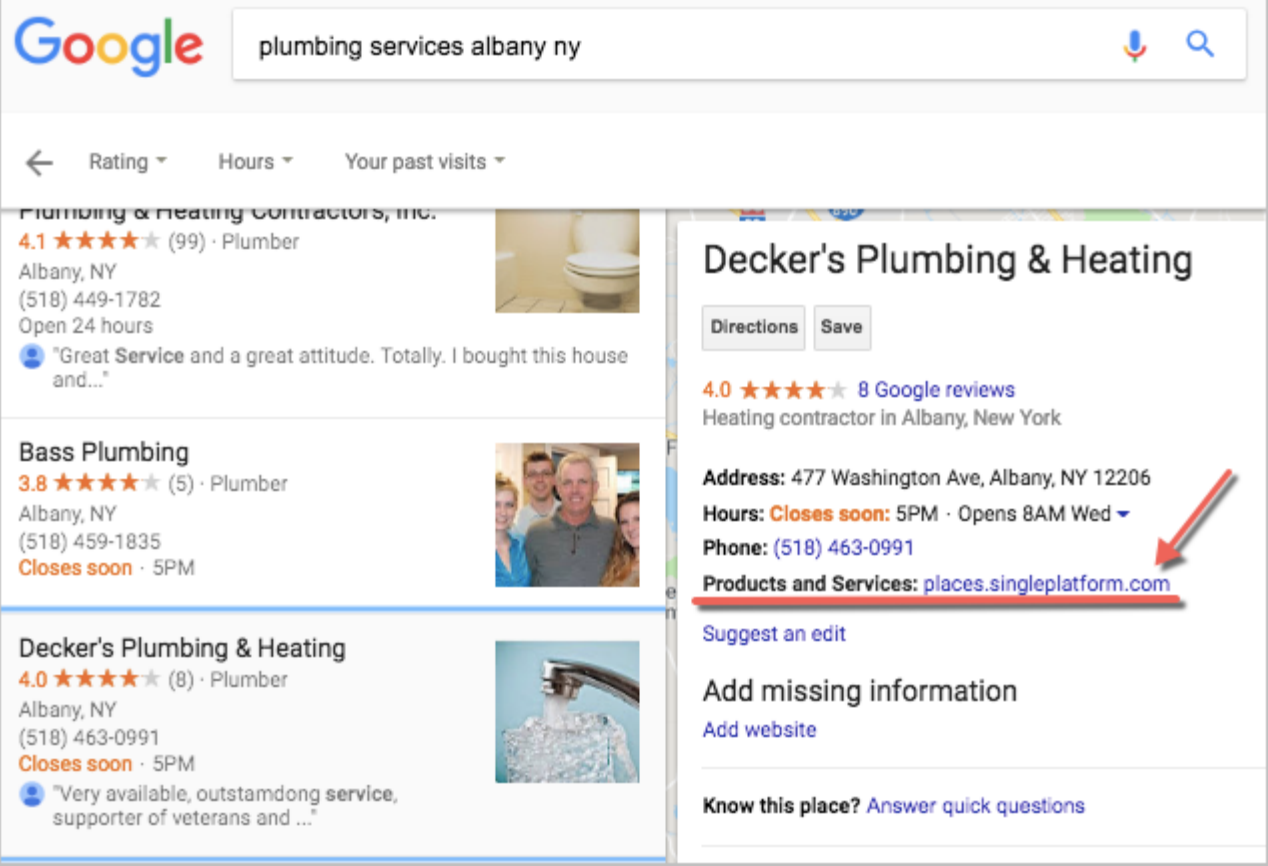Here is the refined and detailed caption for the image:

---

In this detailed screenshot of Google search results for "plumbing services Albany NY," the search box is prominently displayed at the top. 

1. **First Result:** 
   - **Business:** Plumbing and Heating Contractors Incorporated
   - **Rating:** 4.1 stars based on 99 reviews
   - **Location:** Albany, New York
   - **Contact:** 518-449-1782
   - **Hours:** Open 24 hours
   - **Highlights:** Noted for great service and a positive attitude. One review mentions, "I brought this house..."

2. **Second Result:** 
   - **Business:** Bass Plumbing
   - **Rating:** 3.8 stars based on 5 reviews
   - **Location:** Albany, New York
   - **Contact:** 518-459-1835
   - **Hours:** Closes soon at 5 p.m.

3. **Third Result:**
   - **Business:** Deckard Plumbing and Heating
   - **Rating:** 4 stars based on 8 reviews
   - **Location:** Albany, New York
   - **Contact:** 518-463-0991
   - **Hours:** Closes soon at 5 p.m.
   - **Highlights:** Reviews praise its availability and outstanding service, as well as its support for veterans.

On the right side, there’s a highlighted section for Deckard Plumbing and Heating, with information on products and services available at places.singleplatform.com. This is emphasized by a red line underlining it and a red arrow pointing towards it.

---